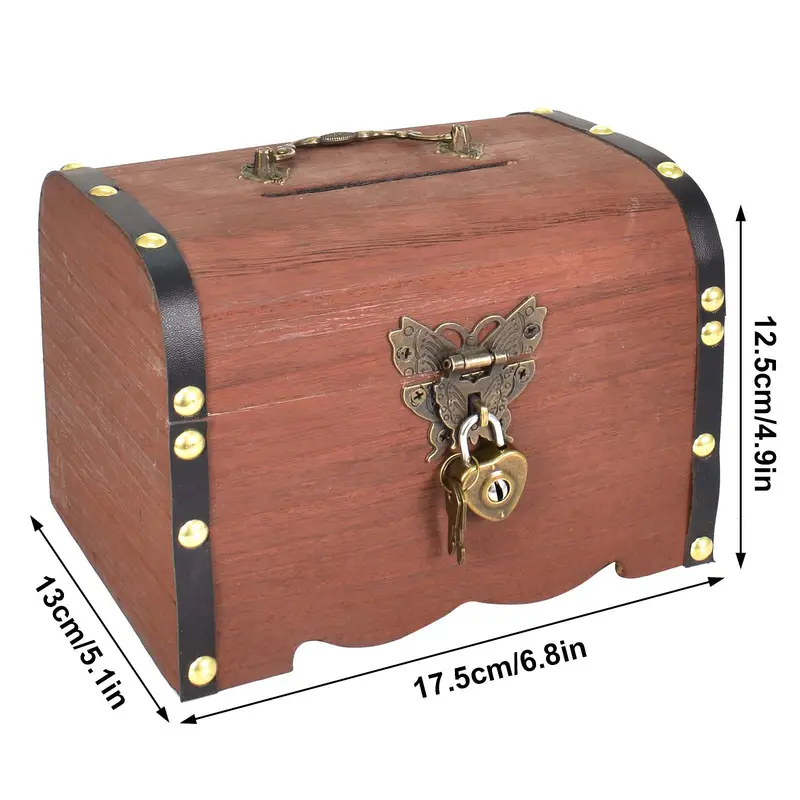The image showcases a vintage-style chest made of brown chestnut wood, featuring a darker brown, almost leather-like, riveted edge. The chest is adorned with gold rivets and a butterfly hinge, which adds to its antique appearance. There's a gold or bronze heart-shaped lock on the front, from which two keys dangle. A gold handle is situated at the top, directly behind a slot designed for dropping items, possibly letters or ballots, into the chest. The chest measures 13 centimeters (5.1 inches) wide, 17.5 centimeters (6.8 inches) long, and 12.5 centimeters (4.9 inches) high. The detailed wood grain and the contrasting black trim give the chest a beautiful, vintage look.